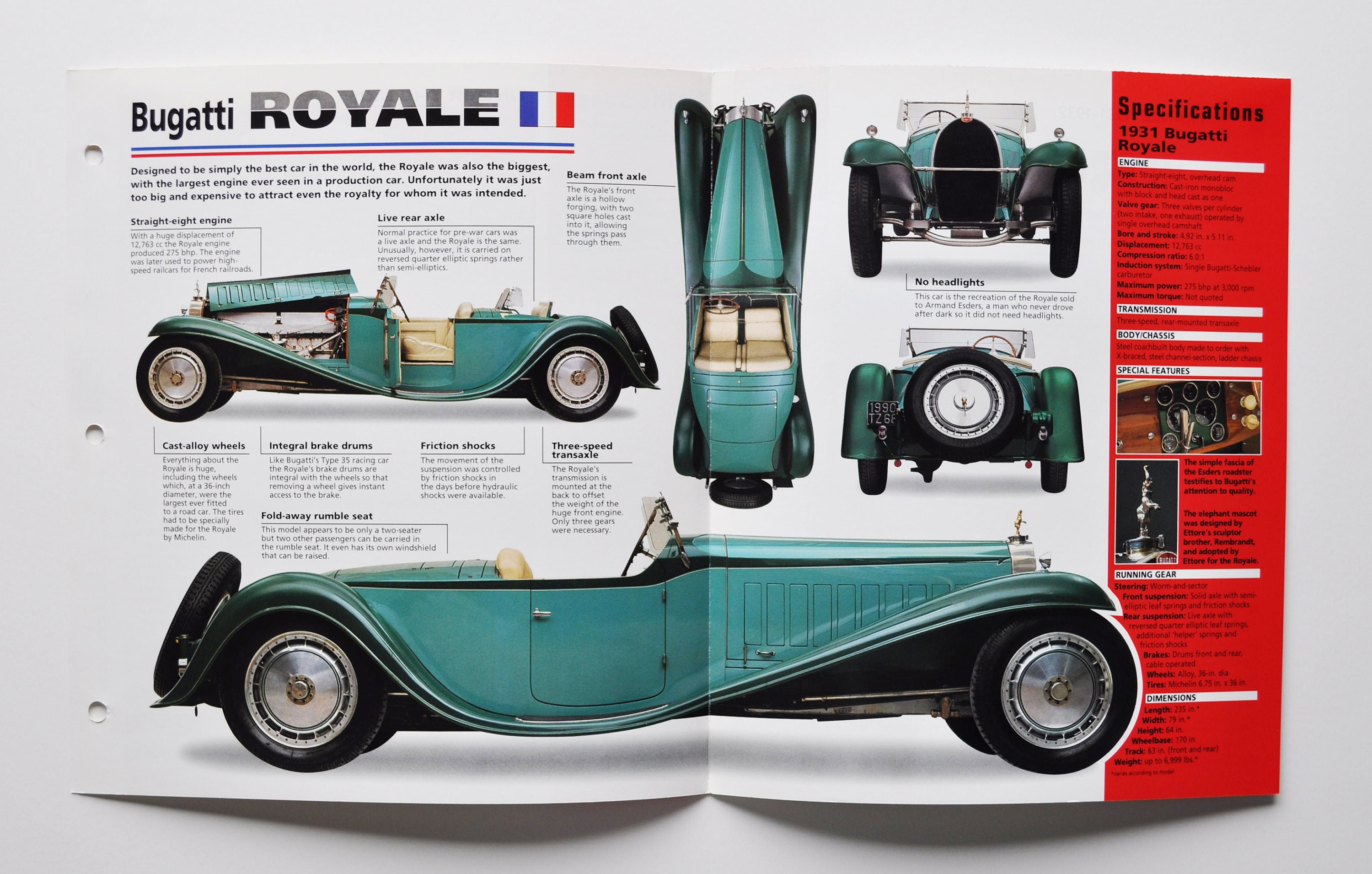The image features an open magazine lying on a white surface. The magazine showcases a vivid photograph of a vintage car, specifically a 1931 Bugatti Royale, in a striking bright green. This elegant vehicle is depicted in multiple views: from overhead, side, back, and front, highlighting its intricate design and sleek, elongated, rocket-like shape. Notably, the car is an open two-seater with no back seat and possibly a trunk, adorned with a spare tire attached to the rear. Prominent bold black letters spell out "Bugatti Royale," accompanied by the French flag on the page. To the right, a vertical red column labeled "Specifications" contains detailed textual information about this classic automobile.